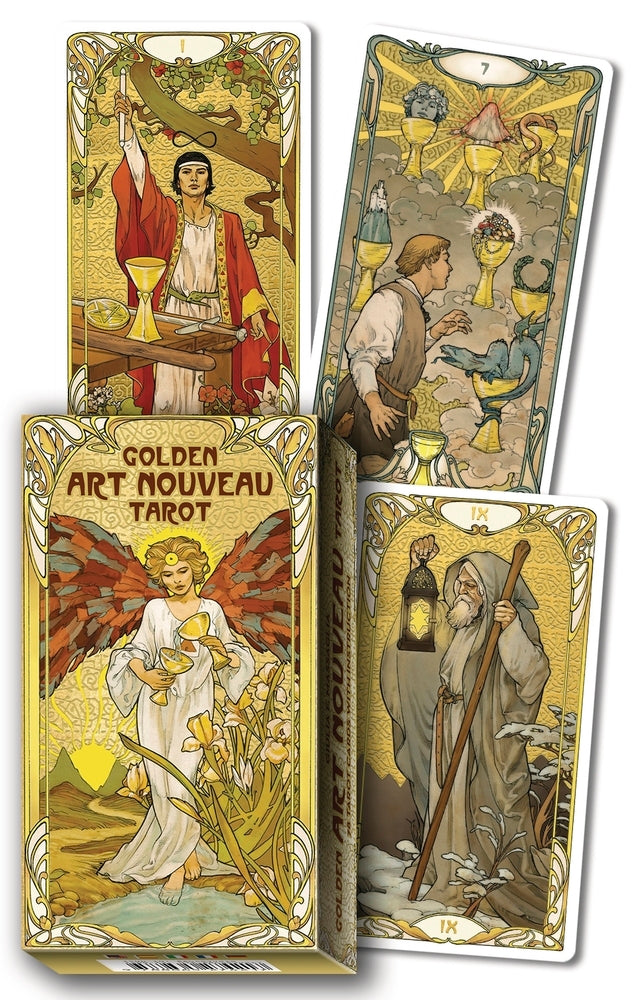The vertical rectangular image showcases a set of Golden Art Nouveau Tarot cards along with their ornate box. The box, positioned at the bottom left, features a 3D computer graphic of an angelic woman in a flowing white robe, holding two goblets and pouring water between them while standing in a stream. Her large, reddish-brown wings are spread wide, and above her, the box is labeled "Golden Art Nouveau Tarot." Surrounding the box are three distinct tarot cards. The top left card depicts a figure in a red robe with a white dress underneath, holding a scroll aloft with various symbolic items—like a golden cup and a sword—arranged on a table before him. To the right of this card, another card presents a man contemplating several golden cups, each filled with different objects, including money and a serpent. At the bottom, there is an old man in a gray cloak, labeled with the Roman numeral IX, clutching a lantern glowing yellow and a large wooden stave, reminiscent of Father Time. The image vividly captures the intricate designs and mystical aura of the tarot set.